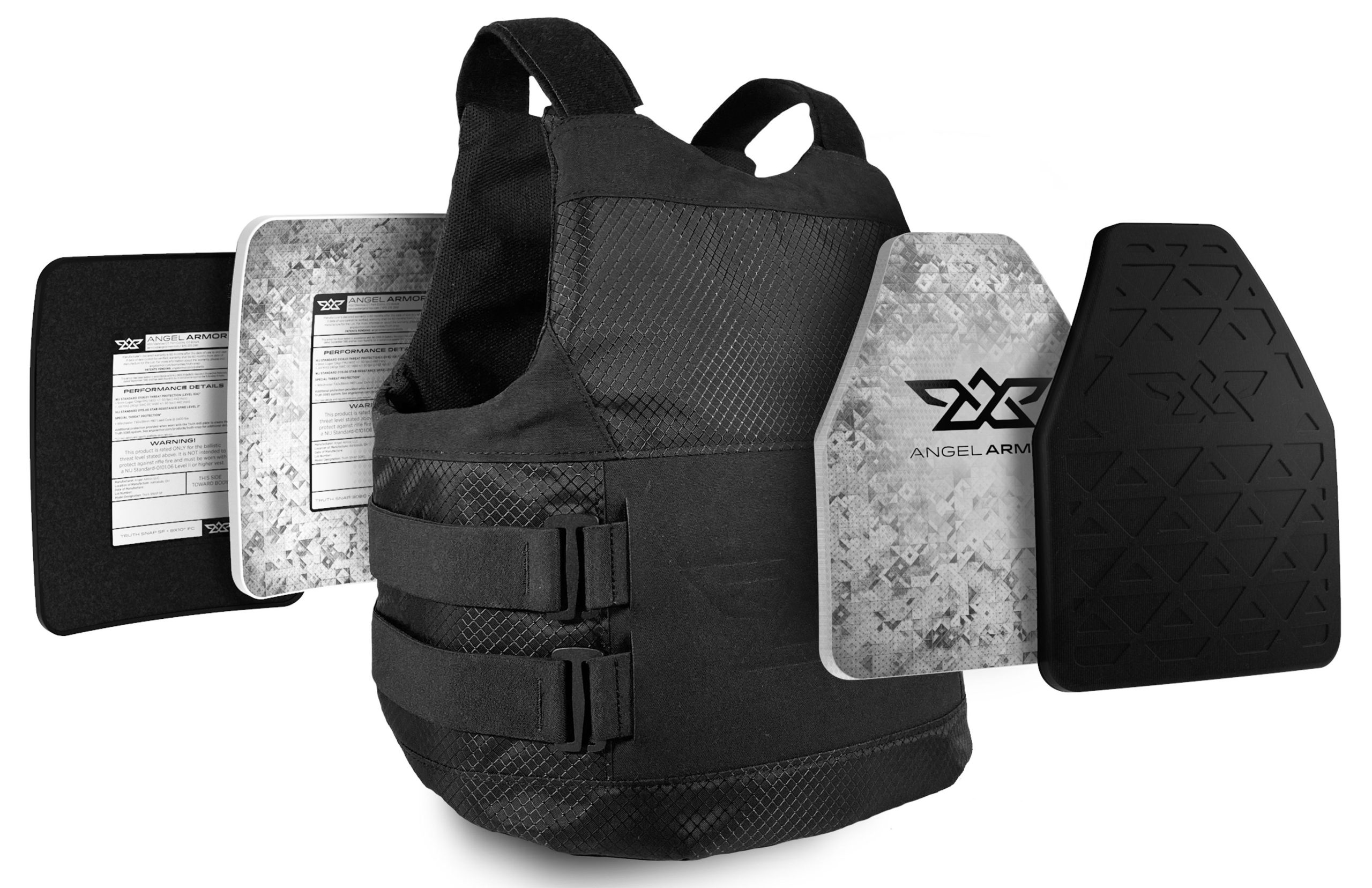The image features a detailed photograph of a black bulletproof vest, prominently displayed against a white background. Central to the composition, the vest is designed with adjustable side straps and shoulder straps, providing a secure fit. On both sides of the vest, there are protective plates showcased: the front plates have a distinctive house-shaped design with triangular patterns, while the back plates are square. These plates are a gray and white fractal pattern, exhibiting the Angel Arms logo—a stylized 'A' with wings extending from the sides. The logo appears embossed on what looks like rubber or plastic mats, also shown on either side of the vest. This comprehensive display includes the Kevlar components, indicating the vest’s bulletproof quality and emphasizing its construction and branding details.